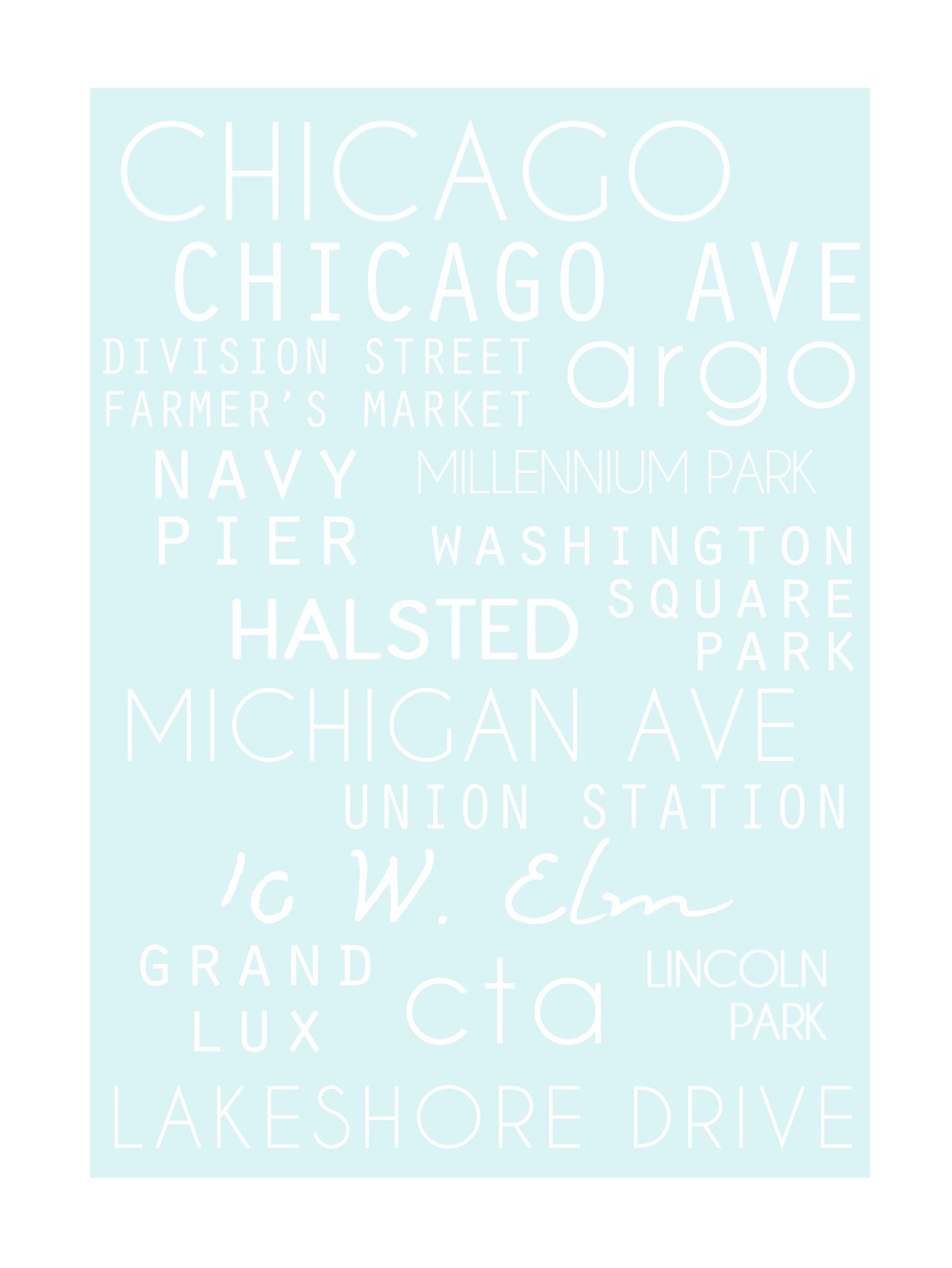The image features a light, teal or mint blue background adorned with an array of street names and significant locations in white text. The names, composed in a script-like format, include prominent Chicago destinations such as Chicago, Chicago Avenue, Division Street, Farmer's Market, Argo, Navy Pier, Millennium Park, Washington Square Park, Halstead, Michigan Avenue, Union Station, Grand Lux, CTA, Lincoln Park, and Lakeshore Drive. An intriguing detail in the list is a script that reads "W. Elm." The repetitive element of street and place names highlights the urban vibe of the city, set against the subtle, pastel-colored backdrop.